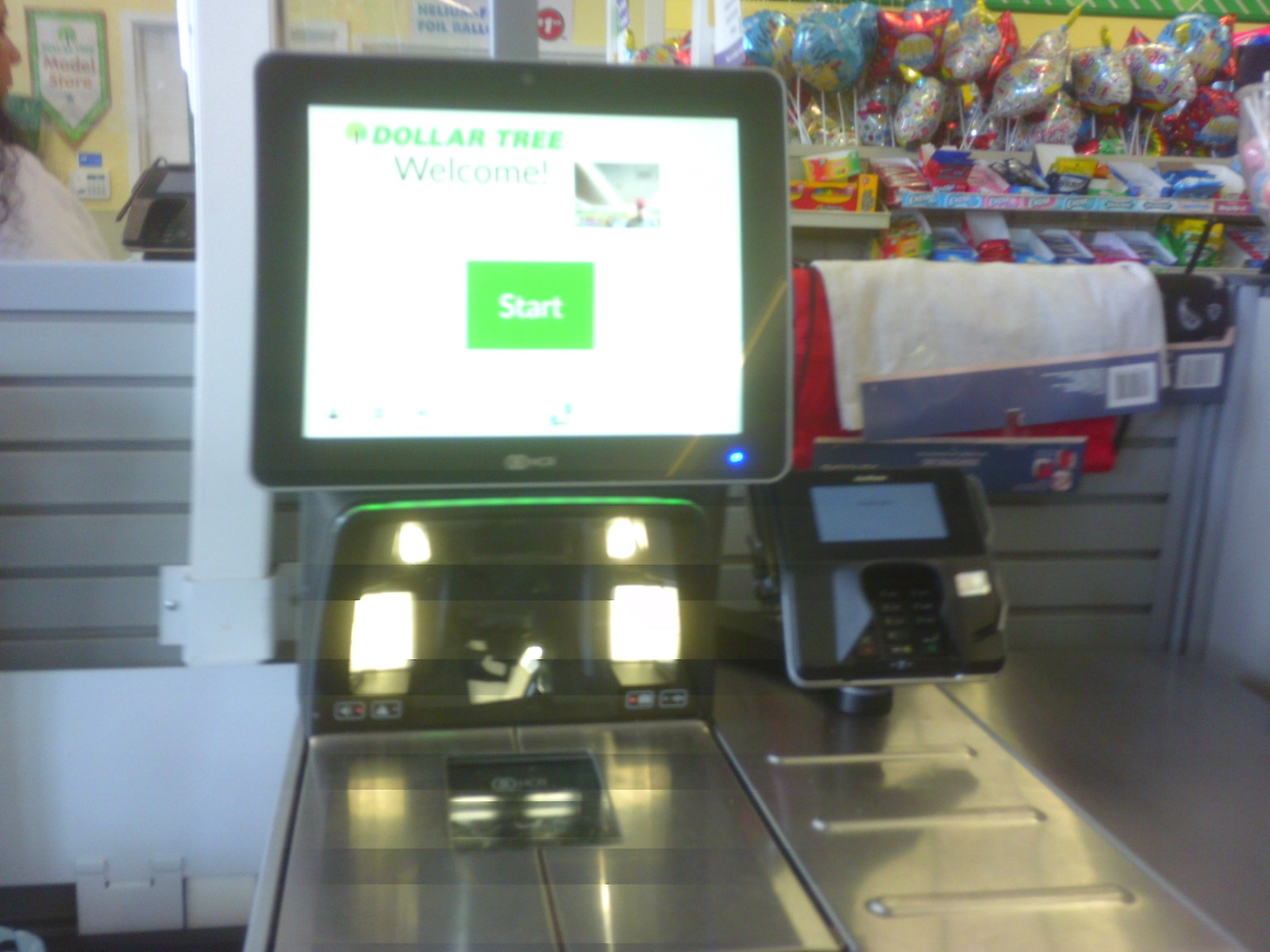This detailed photographic image captures the self-checkout area within a Dollar Tree store. The focal point is a silver checkout stand featuring a computerized monitor displaying the Dollar Tree logo and a large green button labeled "Start" welcoming customers. To the side of the checkout stand, there is a credit card machine and some hanging bags. The setup is illuminated by built-in lights. In the background, shelves stocked with an array of gum, candy, and various party balloons, including birthday balloons, stretch across the space. A wall with a window is visible to the left behind the checkout, through which part of a person—head and shoulders—can be seen, although the text on a sign in the window remains unreadable. Additional elements include towels hanging from the shelves, yellow walls in the background with a white door, and some flags overhead, adding to the store's branded decor. The overall style of the photograph is representational realism, capturing the everyday hustle and bustle of a Dollar Tree store's self-checkout area.